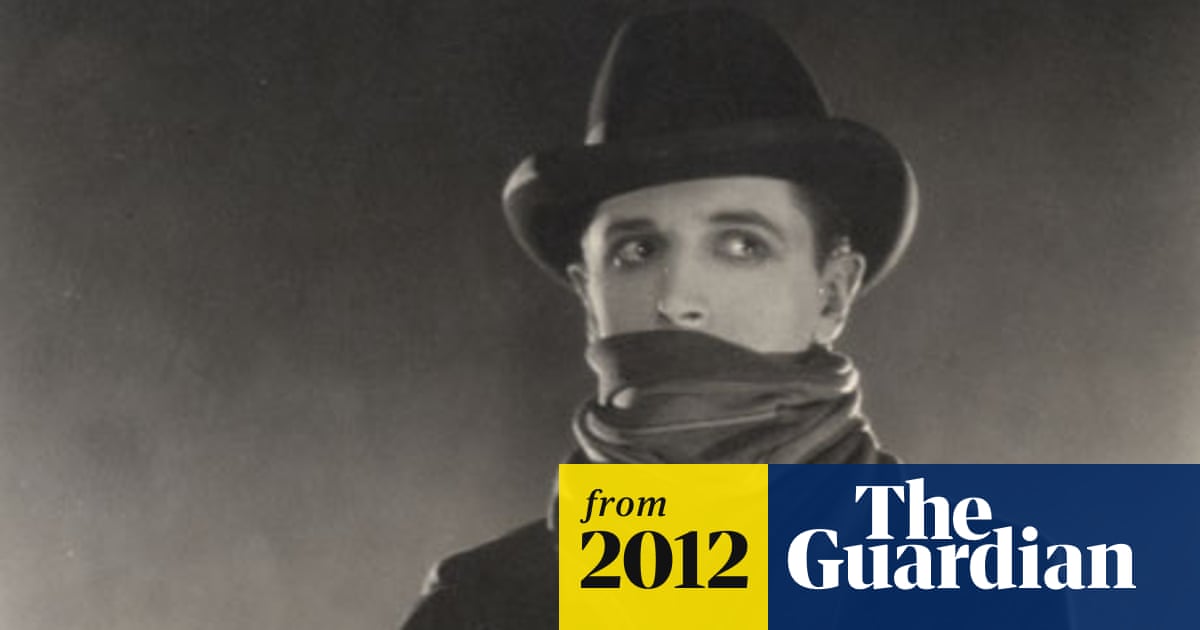The image is a black-and-white photo, possibly from a vintage cowboy movie or show, evoking a sense of the silent film era. It features a man wearing a cowboy hat and a bandana covering his mouth, likely resembling characters such as the Lone Ranger. He is facing slightly to the left while his gaze is directed to the right, suggesting he is observing something. The man is dressed in a dark jacket, though the black-and-white format obscures finer details. The background is smoky, transitioning from darker at the top to lighter at the bottom. In the lower right corner, two rectangles appear: a yellow one with black text reading "From 2012" and a blue one with white text stating "The Guardian," indicating that the image is part of an advertisement or feature related to The Guardian from 2012.